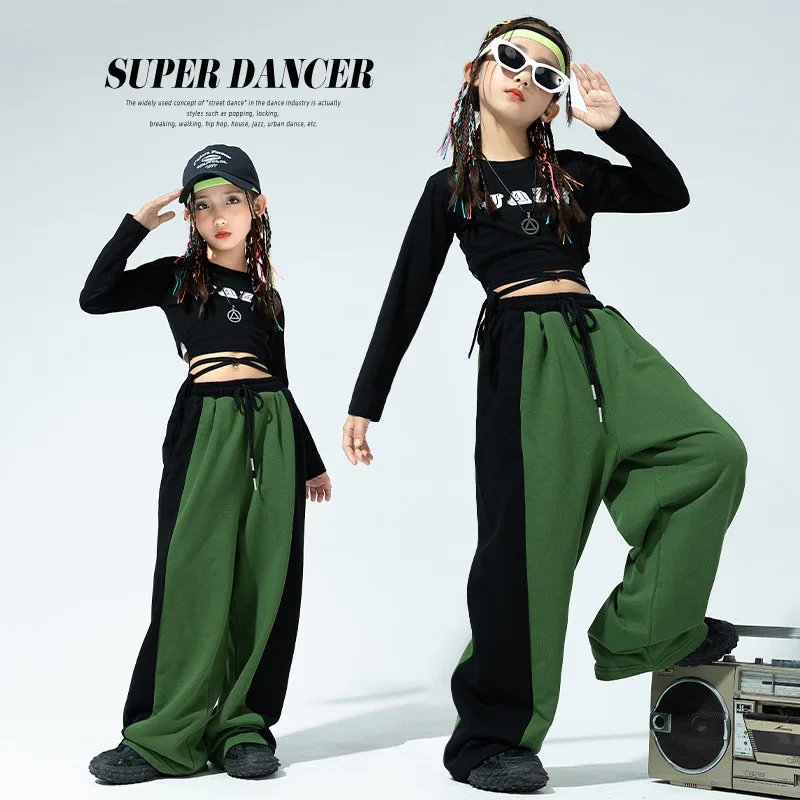This image is an advertisement for "Super Dancer" and features two young Asian girls, approximately 7 to 10 years old, giving off a hip hop vibe. The text "Super Dancer" is prominently displayed at the top in black. On the left side, one girl is wearing a green bandana around her forehead, a hat, green baggy pants, and a stylish black top that exposes her midriff. She has colorful ribbons braided into her hair and sports a distinctive necklace with a circle and triangle in the middle, completing her look with black shoes. Standing on the right side is the same girl, now posed on a boom box. This time, she's without the hat but wears a white pair of sunglasses and a bandana, maintaining the same green and black outfit. Both girls have matching black tops with some writing, baggy pants with strings hanging from them, and are accessorized with braids and unique necklaces. With their dynamic pose and attire, the girls exude a cool, urban dance style, emphasizing hip hop culture and fashion.